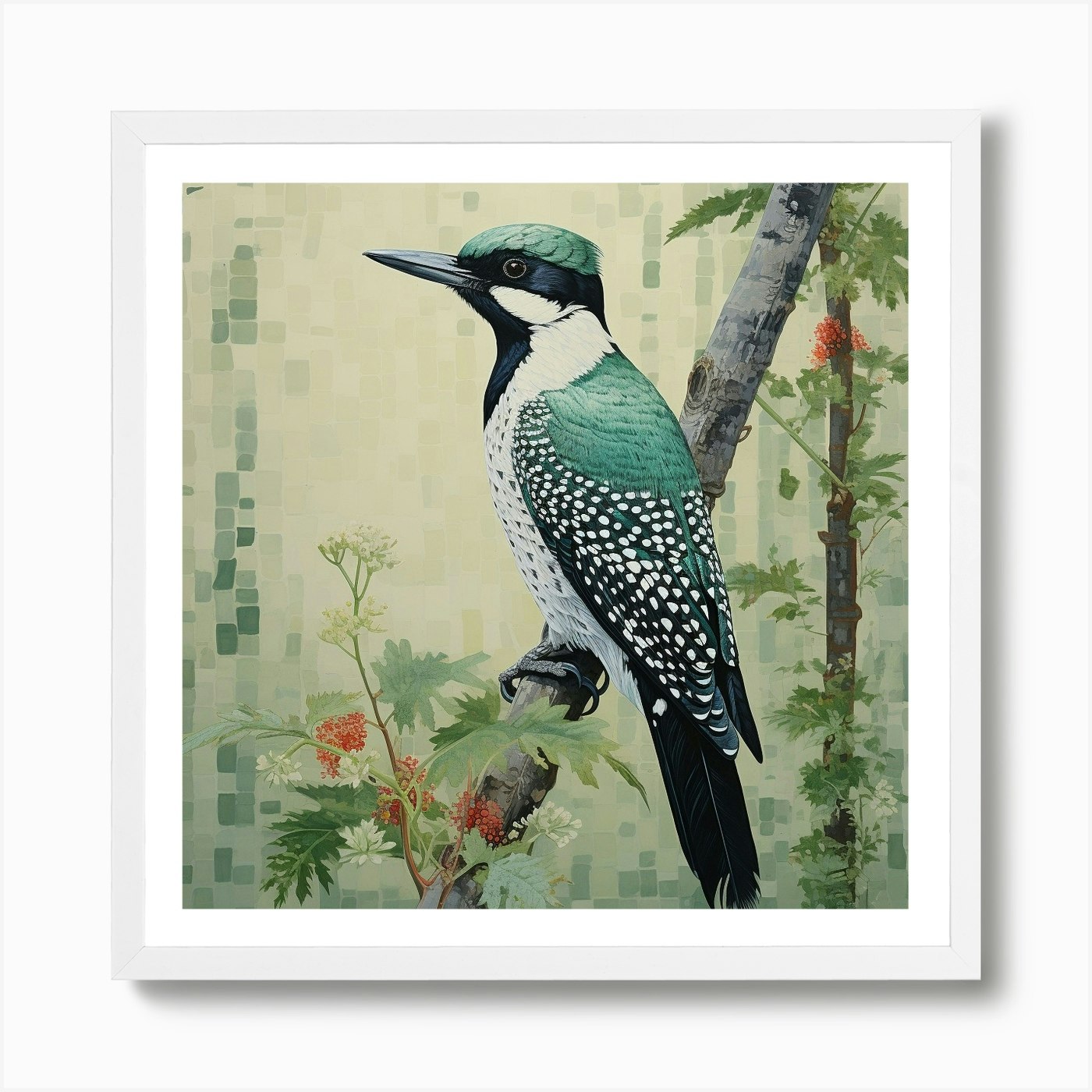In this detailed watercolor painting, a vibrant woodpecker takes center stage, perched on a realistic-looking gray tree branch that begins horizontally before curving upward. The woodpecker's talons grip the branch firmly, lending a sense of immediacy and life to the artwork. Its plumage is a striking blend of colors: a green crown and shoulders, with black extending over its eyes and neck, merging into a black tail. The wings are dominantly black, flecked with white dots, and the underparts are predominantly white with scattered black spots. The bird’s throat and beak are distinctly black, adding to the sharp focus of the bird itself, which contrasts with the softer, more abstract background. The backdrop is composed of delicate, muted gray-blue squares interspersed with a small tree adorned with green leaves and pale red berries. Below the bird, additional details such as white flowers, red berries, and green leaves introduce subtle accents, harmonizing with the greens of the woodpecker’s feathers. The background maintains a neutral, off-white hue, which enhances the composition’s overall balance.